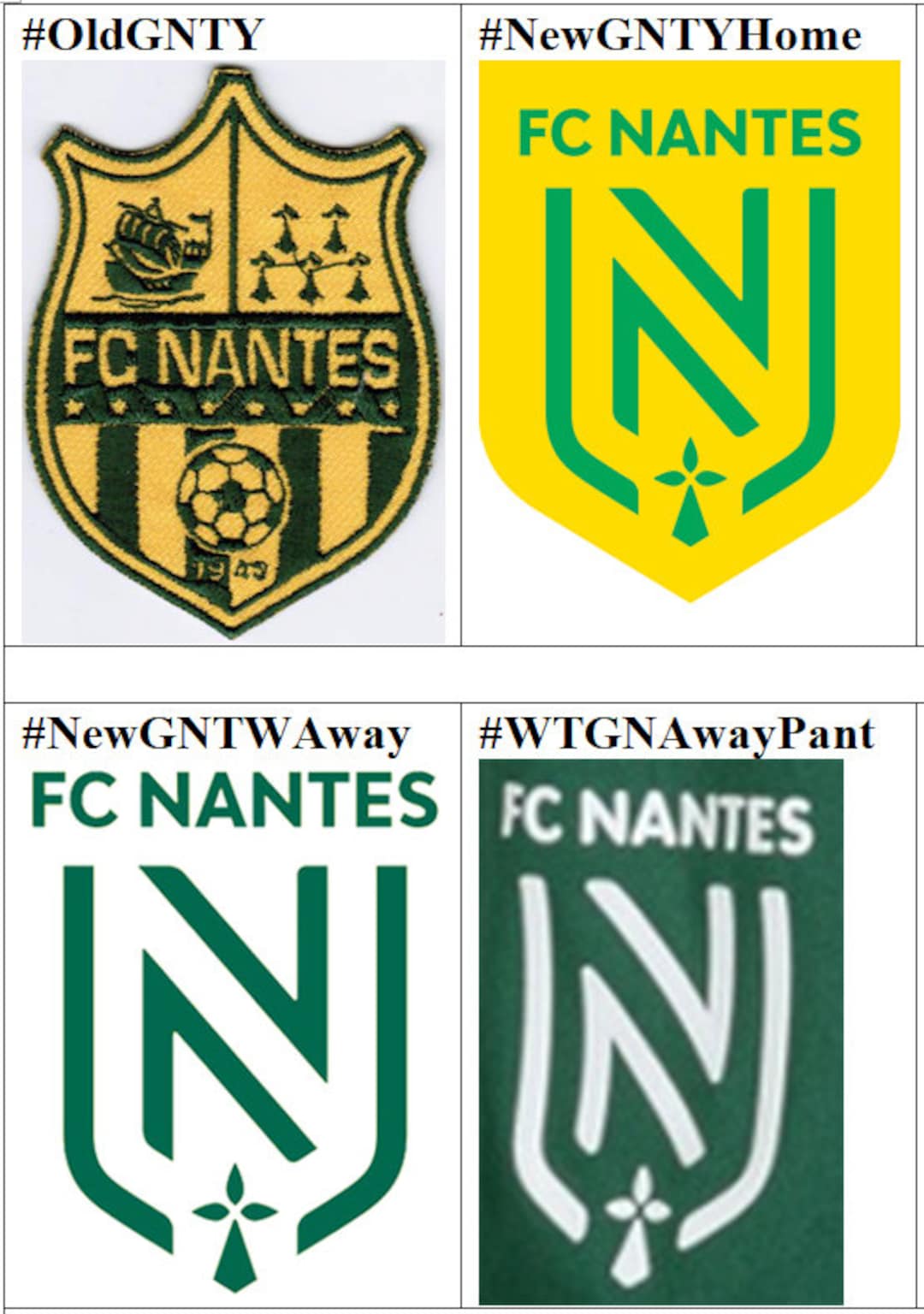The image showcases a comparison of four different FC Nantes logos, arranged in a four-square grid. In the top-left corner, there is an old, very old, logo designed to resemble a physical badge, featuring a clipper ship, a soccer ball, and what appear to be five lighthouses. This logo is accompanied by the hashtag #OLDGNTY and a black text label at the top. Adjacent to it in the top-right corner, is a digitally simplified version of the logo with a yellow background, green tree leaves, and the FC Nantes name prominently displayed at the top.

On the bottom-left, the logo is presented without a backdrop, consisting solely of the typography, and is tagged with #NEWGNTYAway. Lastly, in the bottom-right corner, the logo features FC Nantes lettering in white ink set against a green background, and is associated with the hashtag #WTGNAwaypaint. Each logo iteration provides a distinctive look and feel, capturing the evolution and different stylistic approaches of the club’s branding.